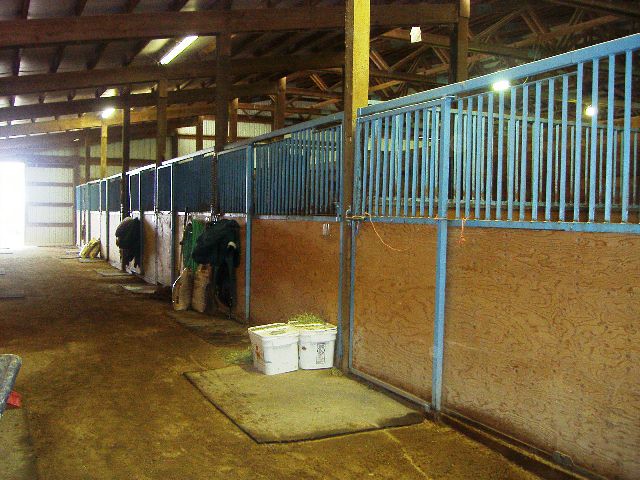This photograph captures the interior of a horse barn with multiple stalls. The stalls are structured with wooden panels at the bottom and light blue metal bars on top. The floor has a yellowish-tan, worn-out appearance. Hanging in and around the stalls are various items, including green jackets in the middle stall and possible equipment. In the foreground, there's a pad and two white tubs containing hay. The wooden ceiling features supporting beams, contributing to the barn's rustic aesthetic, with some fluorescent lights visible overhead. At the far end, the open barn door lets in a flood of bright light, though the exterior details are obscured by the brightness.